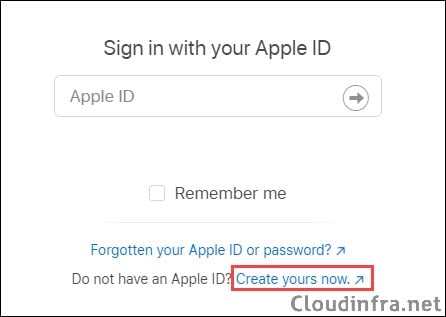The image depicts a portion of an Apple ID sign-in interface. At the bottom, there is a red rectangular outline around the text "Create yours now." This text, along with a blue arrow pointing to the upper right-hand side, indicates a clickable hyperlink. The phrase "Create yours now." is positioned to the right of the question "Don’t have an Apple ID?" Above this, another blue hyperlink reads "Forgotten your Apple ID or password?" accompanied by an upward-pointing arrow. Further up, there's the text "Remember me" next to an empty checkbox. Above the checkbox, there are two spaces above which lies a text input box labeled "Apple ID." The directive "Sign in with your Apple ID" is situated above the text input box.